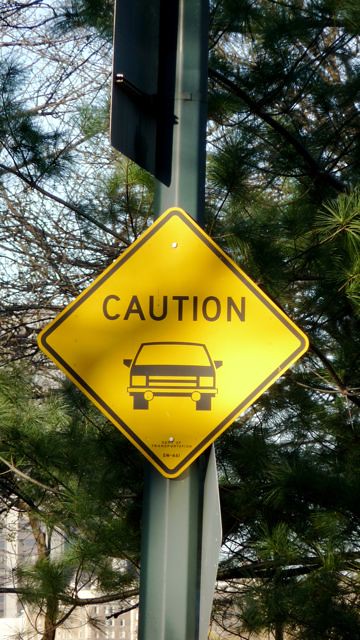This is a close-up photograph of a caution sign mounted on a dark green metal pole. The pole extends vertically from the bottom edge to the top edge of the image. Attached to the pole, facing away from the camera, is the barely visible backside of another sign. Prominently displayed in the center of the photo is a yellow, diamond-shaped caution sign bordered in brown, with the word "Caution" in black print. Below the text, there is a simple brown outline of a car driving towards the viewer. 

The background is dominated by treetops and branches, primarily an evergreen tree with needle-like leaves and some bare patches at the top, allowing glimpses of a bluish-gray, cloudy sky. There's also a mix of other tree branches and green leaves covering a significant portion of the background. The setting feels open, as if on a street or roadside, with the natural elements providing a textured backdrop to the caution sign.